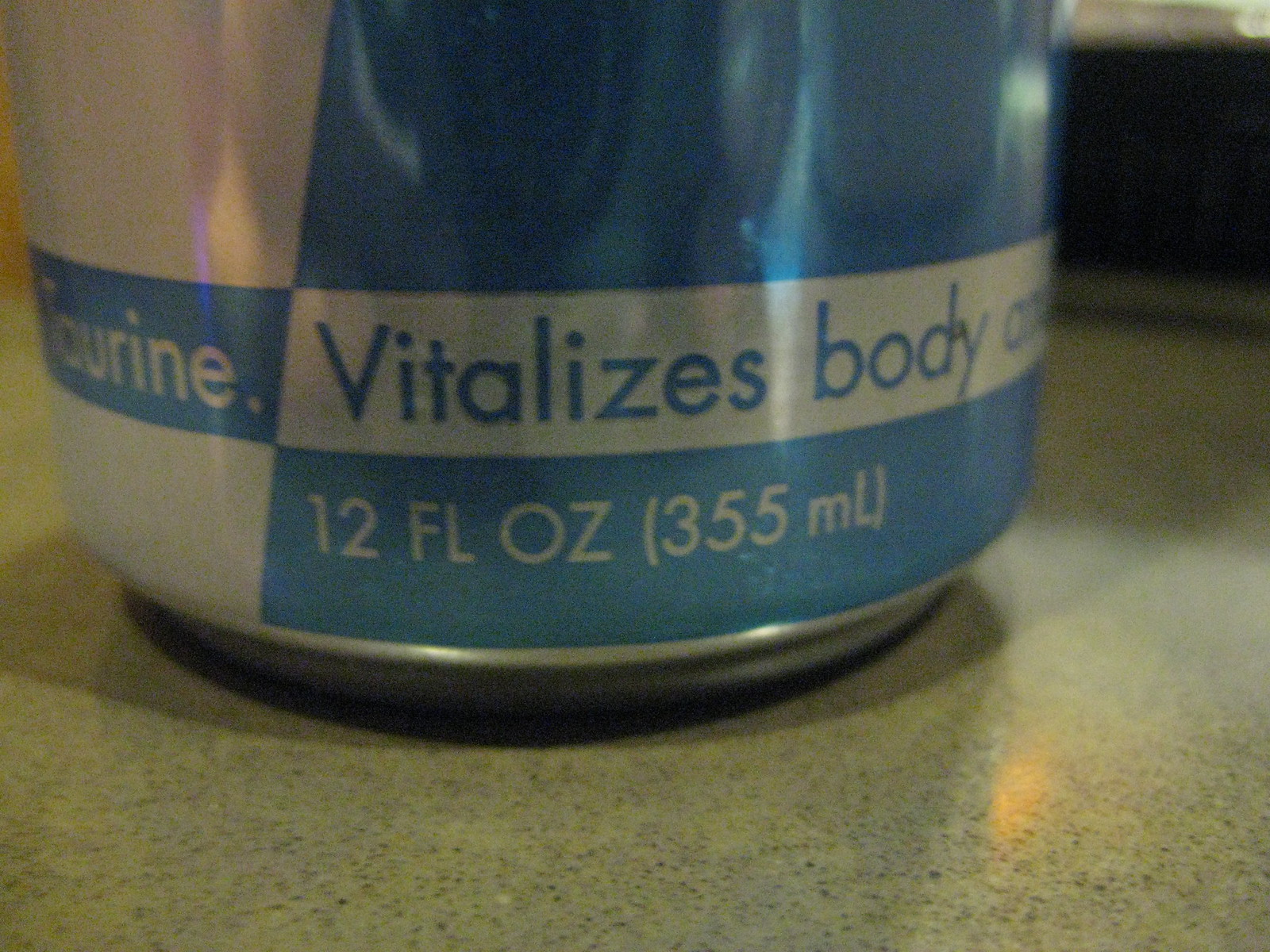**Close-Up of an Aluminum Can on a Laminate Counter**

In this close-up image, an aluminum can, which seems to have a design reminiscent of a soda can, is prominently featured on a light gray laminate counter speckled with dark gray. The can exhibits a visually striking combination of light to medium blue and white colors, with the blue areas possessing a reflective quality that captures and mirrors the ambient light in the room. 

The can is positioned with blurred brown elements visible in the background on the right, suggesting possibly wooden objects or cabinetry in out-of-focus areas. On the upper left section of the can, a large white area is present, beneath which lies a smaller blue rectangle with partially legible text that reads "T-O-U-R-I-N-E." It's uncertain if additional letters precede this segment.

Further down, another longer blue rectangle contains the phrase "vitalizes body," though the succeeding word is indistinguishable. Below this, informational text denotes the can's volume as "12 FL OZ" followed by its metric equivalent in parentheses "(355 ML)."

Additionally, there is a notable golden reflective spot on the counter surface beside the can, further emphasizing the interplay of light within the scene.